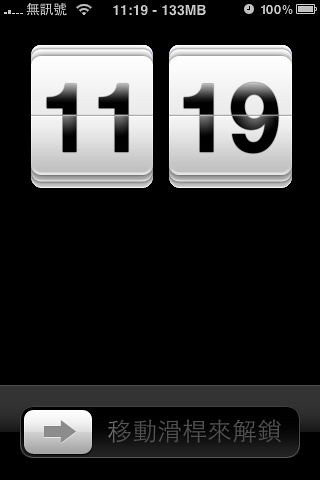This rectangular image, oriented vertically, appears to be a screenshot taken from a smartphone. The background is entirely black, providing a stark contrast to the white and gray elements displayed on the screen. 

Starting from the upper left corner, the signal strength indicator is shown in the form of bars progressing from left to right. Adjacent to this are some characters resembling Chinese text, followed by a Wi-Fi signal strength icon. Moving towards the center, there is a digital readout displaying "11:19 - 133 MB" in white text. The right-hand corner of this upper section contains a clock symbol that reads "100%", accompanied by a fully charged battery icon beneath it. 

Dominating the upper portion of the image is a large, prominent timestamp, showing "11:19" in bold white font. The writing within this timestamp is black, offering a clear and distinct look. 

At the bottom of the image, there is a sliding arrow feature, likely to unlock the phone. The base of the arrow is white, while the arrowhead itself is gray. To the right of this arrow, there are additional Chinese characters.

Overall, the image captures a typical smartphone lock screen interface with clear indicators for signal, time, battery life, and a slide-to-unlock feature, all set against a black background which enhances the readability of the white and gray elements.